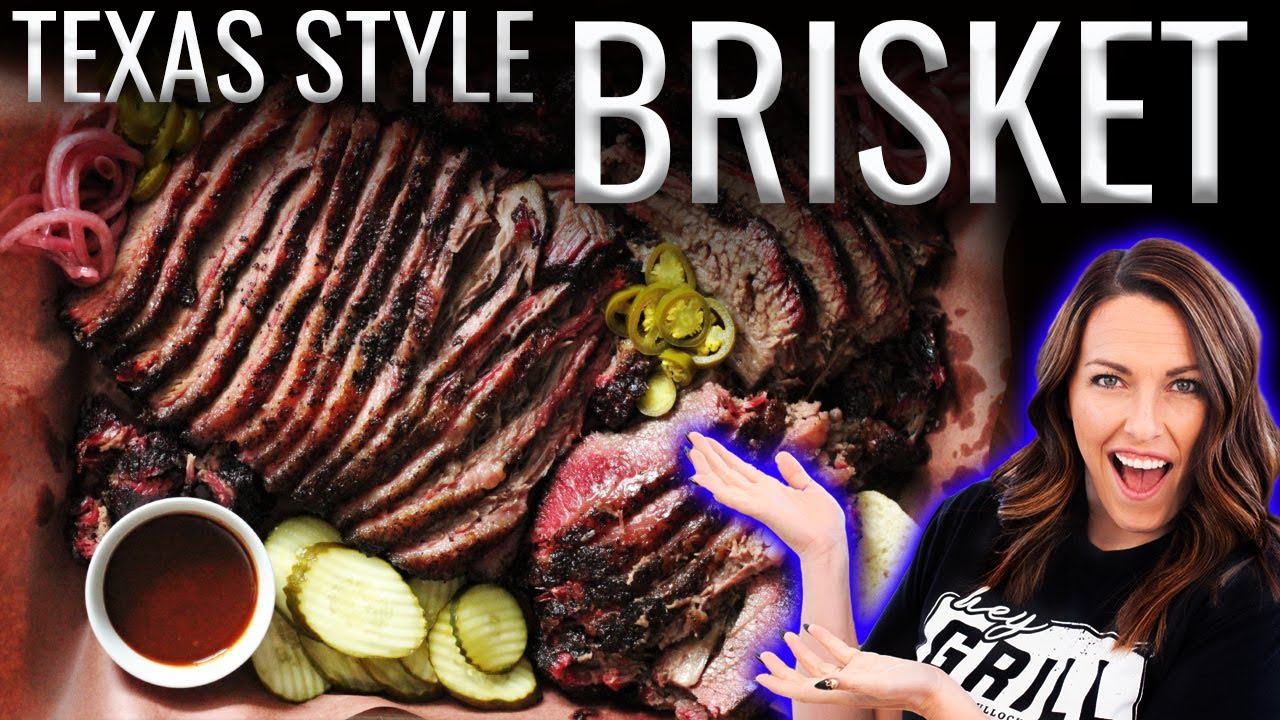The image showcases an ad prominently displaying "Texas Style Brisket" in bold white text at the top. Dominating the left side of the image is a mouthwatering sliced brisket arranged in a formation that gives a sense of depth and abundance. The tender, juicy brisket is garnished with tiny pickle slices and jalapenos, adding vibrant pops of green, alongside pickled onions. Nestled in the corner of the dish is a small white container filled with rich barbecue sauce, enhancing the savory presentation.

To the right, a cheerful woman is depicted with a big smile, her white teeth beaming with excitement. She has shoulder-length wavy brown hair and is wearing a black t-shirt that prominently features the logo "Hey Grill." Her hands are raised in a gesture of presentation, highlighting the delicious brisket. She is positioned in the bottom right corner, her figure outlined in a neon-like purple or blue hue, which makes her stand out. She also has long stiletto-style nails with black tips, adding a touch of flair to her look. Her presence, combined with the artful layout of the brisket, creates a dynamic and engaging advertisement.